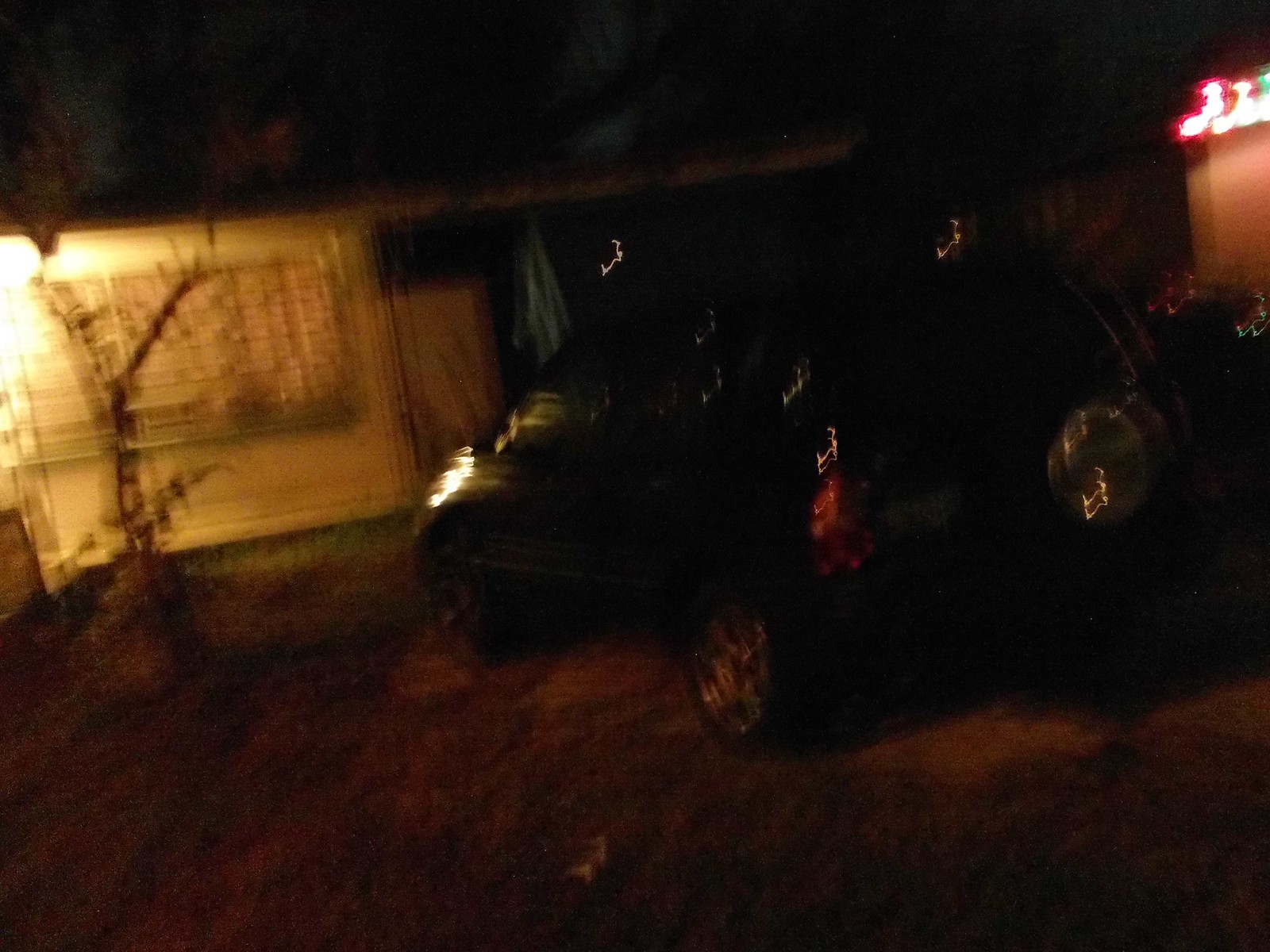A nighttime photograph, slightly blurry, captures two cars parked in the driveway of a single-story home. The house features white siding, a prominent window towards the left side of the front facade, and a brown-colored door. A light is visibly on at the corner of the house, illuminating the surroundings faintly. In front of the house stands a small, bare tree, offering minimal foliage. In the driveway, a black SUV is noticeable, parked on a patch of dirt where the grass has seemingly worn away amidst an otherwise grassy yard. The SUV has a spare tire attached to its rear. Next to the SUV, the outline of another vehicle is discernible as light reflects off its surface.